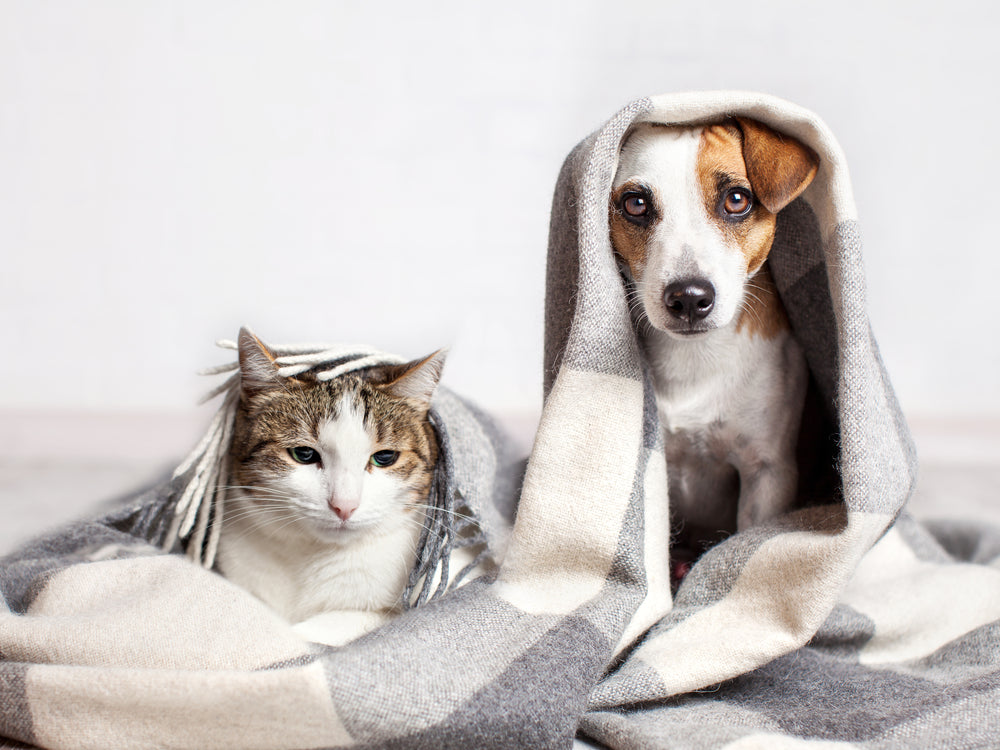In this image, a cat and a dog sit side by side with an air of sluggishness as they face the front. The cat, positioned on the left, has a white face and chest with brown ears, and is partially hidden under a cozy blanket featuring a rectangular pattern in white, light grey, and dark grey. Tassels from the blanket hang over the cat's head, adding a touch of whimsy. The dog, seated on the right, displays a distinct facial marking with a white face center framed by brown sides and a drooping brown ear. Both animals share similar color patterns and are snugly covered by the shared blanket. The background of the image is a clean white, with hints of grey on the wall, enhancing the cozy and intimate setting of the photograph.